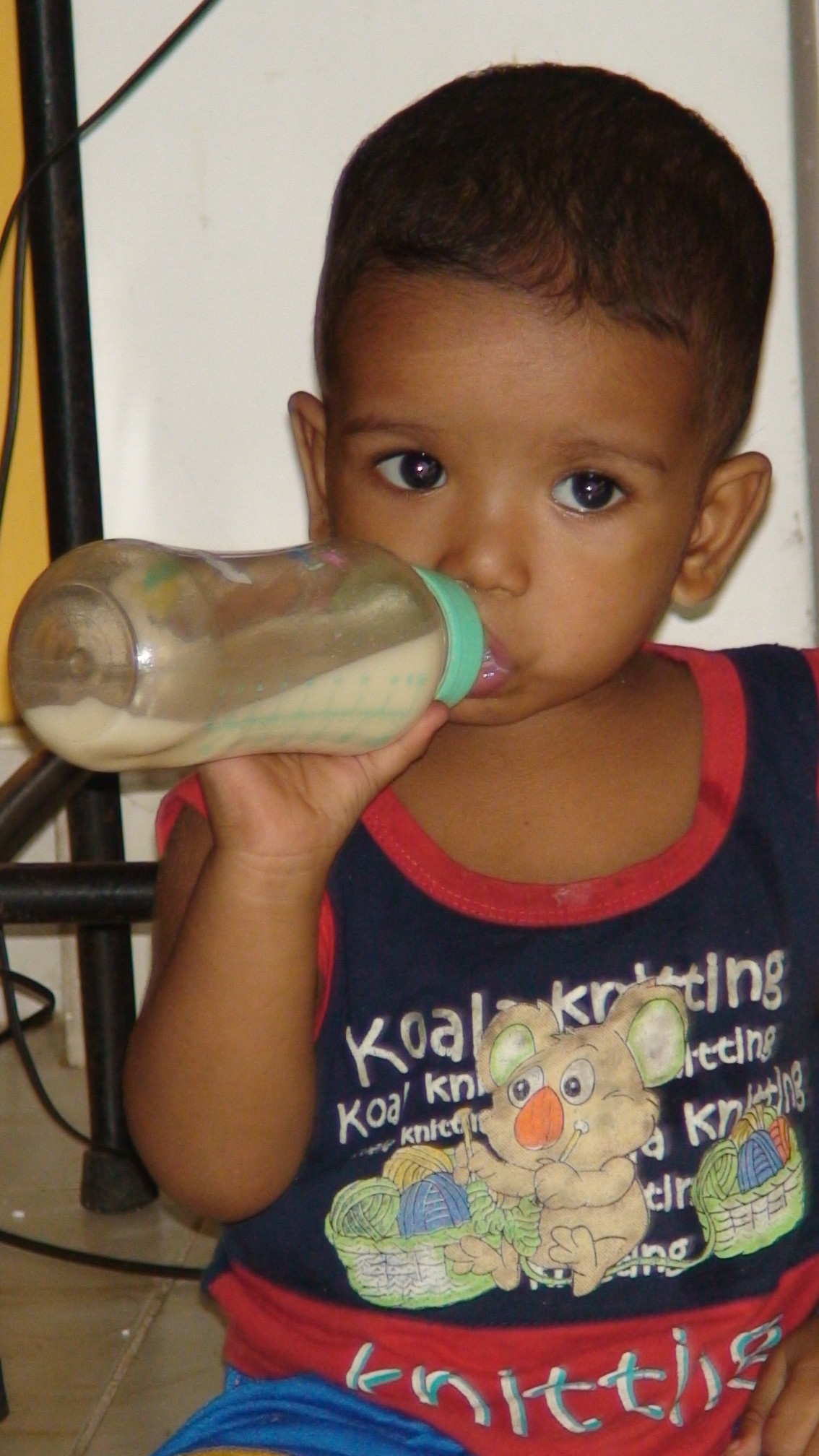In the image, a young boy, approximately one to two years old and with short black hair, is featured. He appears to be darker-skinned and might be of Indian descent. The boy is framed sitting on a beige stone or tile floor with brown streaks. Dressed in blue shorts and a sleeveless tank top that has a blue top and a red bottom, his shirt features a playful illustration of a koala bear knitting, complete with yarn in a green basket, knitting needles, and the words "Koala Knitting".

The child is engrossed in drinking milk from a plastic bottle with a green cap, which he holds up to his lips with his right hand. The bottle is about half full. Behind him, a white wall with yellow hues serves as the backdrop. To the left, there appears to be something orange, possibly a curtain. Also visible is what seems to be a metal stand or chair with thin black legs and horizontal bars. A black cord hangs out of view, hinting at something plugged in nearby. The boy's large head relative to his body and his off-camera gaze suggest he might be looking at something or someone, perhaps his mother.